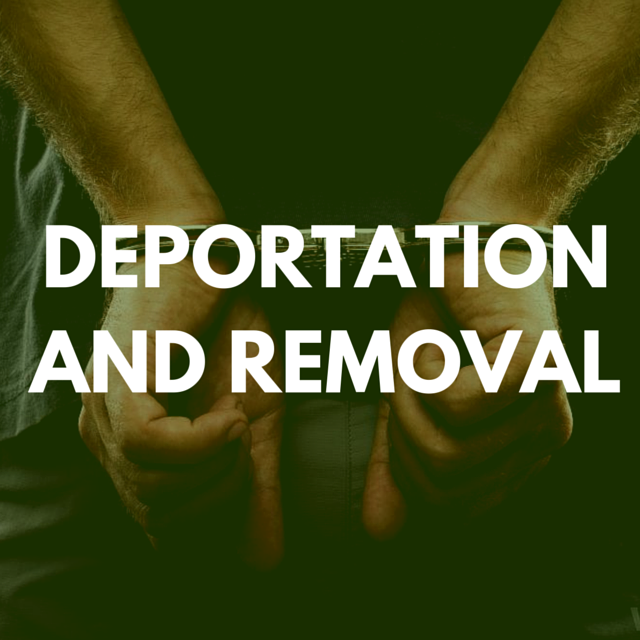This square, slightly faded photograph with a greenish tint captures the image of a person from the back, whose light-colored, hairy arms are handcuffed behind them. The individual wears a black t-shirt and grey pants, blending somewhat into the dark background. White, all-capitalized text overlays the center of the image, reading "DEPORTATION" on the top line and "AND REMOVAL" directly beneath. The text is positioned prominently over the handcuffed hands, emphasizing the restrained state of the person in the photo.